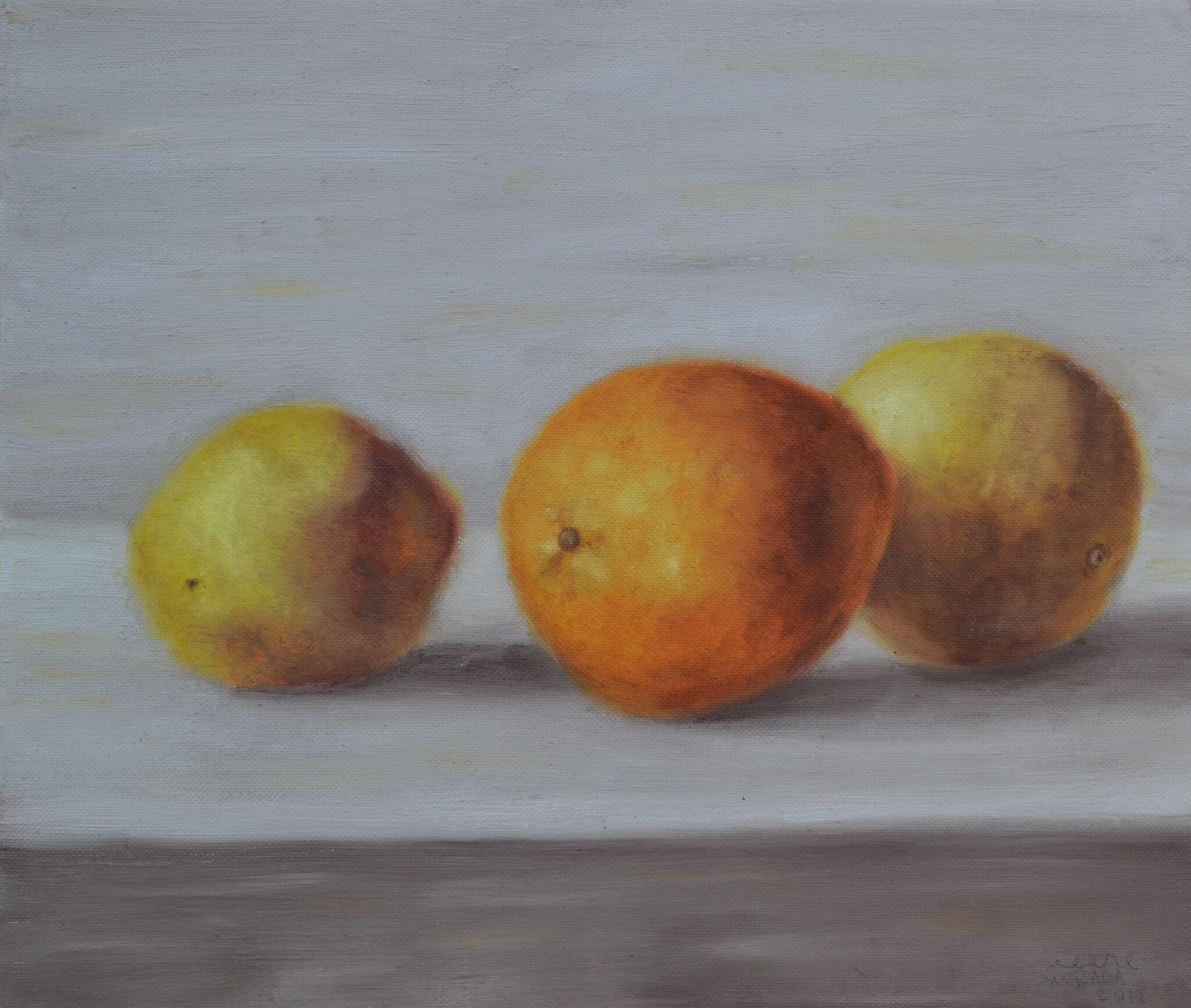The artwork appears to be an oil painting in the style of the masters, depicting three pieces of fruit resting on a surface. The background is a gradient of gray tones, transitioning from a darker shade to a lighter shade, which could suggest a tabletop or counter. The fruit arrangement includes a lemon on the left, an orange in the middle, and an ambiguous round fruit on the right with a yellowish hue but an unclear shape. The painting captures a close-up segment, with soft, dark gray shadows extending to the right, providing a sense of depth. The image exhibits a slightly blurry and grainy texture, reinforcing its description as a painting rather than a real-life photograph. The detailed rendering and use of light and shadow evoke a sense of realism despite the impressionistic blur, highlighting the fruits' vivid colors against the muted gray backdrop.